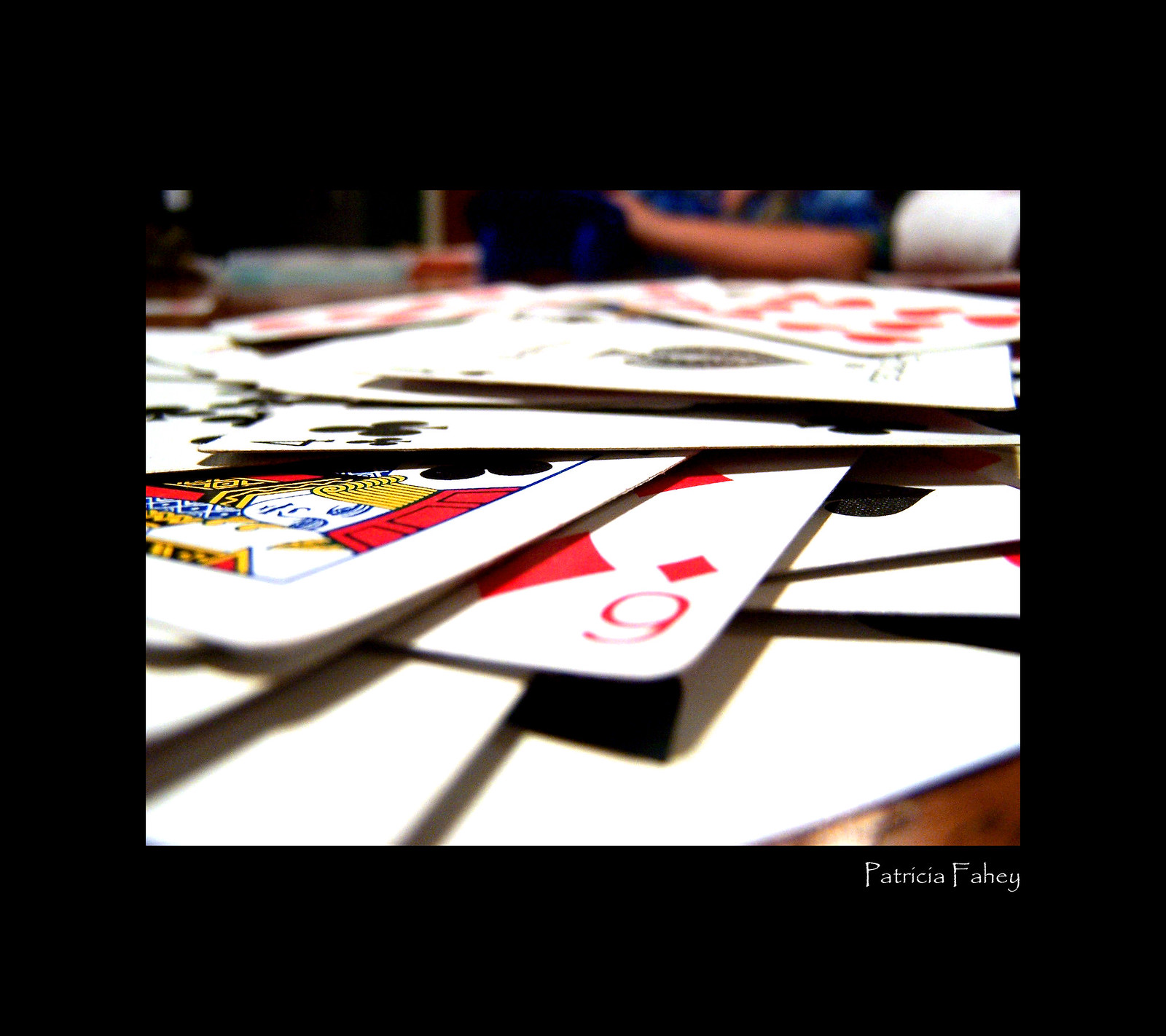This photograph showcases a close-up view of a scattered arrangement of playing cards, significantly overlapping each other. Despite the overlap, a few cards are discernible: a six of diamonds and a jack of clubs prominently appear in the foreground. In the background, an ace of spades and a nine of hearts can also be seen. The image features a digital black border, which gives it the appearance of a poster. The setting is a casual living room, with a dimly outlined person and their arm visible behind the tabletop where the cards are spread. The photographer, Patricia Fahy, has managed to capture an intimate and spontaneous domestic moment.